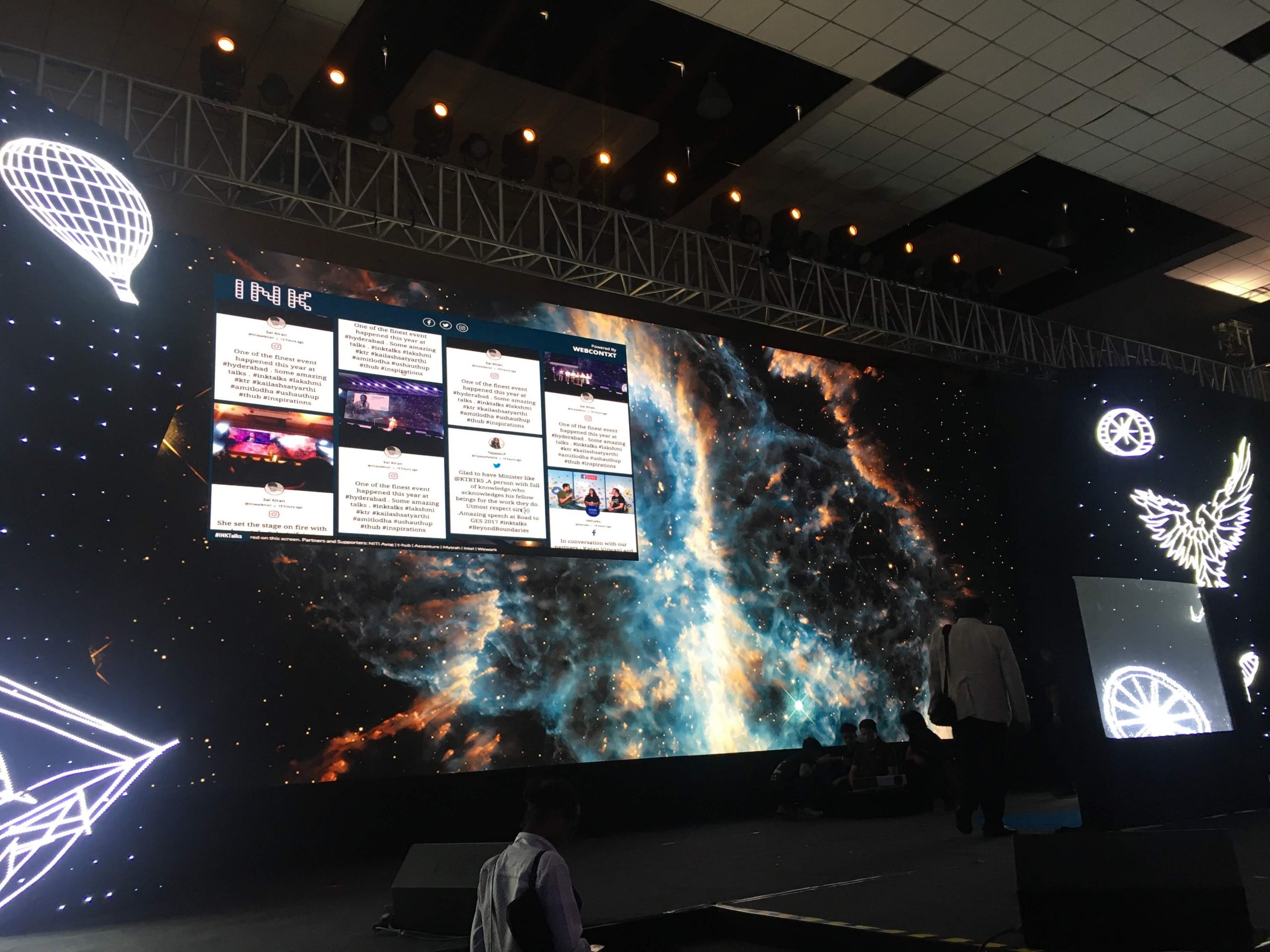This image captures the interior of a spacious convention center with a high ceiling and a stage setup. A striking, enormous LED screen is positioned at the back of the stage, depicting a cosmic scene featuring a galaxy in blue, white, orange, and black hues surrounded by stars. The top left of the screen displays a rectangular computer-like interface titled "ink," featuring social media logos like Facebook, Twitter, and Instagram, alongside unreadable posts or tweets. To the left of the screen, there's an LED symbol of a hot air balloon, and to the right, an LED symbol resembling a phoenix or eagle. Overhead, a metal framework supports the structure, complemented by a white tile ceiling. In the foreground, people are both seated and walking across the stage, contributing to the dynamic atmosphere of the convention.